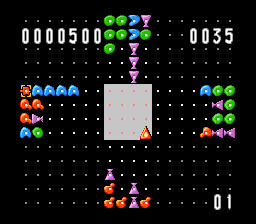The image is a still from an arcade or computer game featuring a black background with a grid of evenly spaced white dots. In the center of the grid, there is a pale grey rectangle filled with neatly arranged red dots. A red triangle sits in the bottom right corner of this grey rectangle. The game screen includes several counters: the top left displays "0000500," the top right shows "0035," and the bottom right corner reads "01." Surrounding the grey rectangle are various colored characters and symbols: round green circles with white centers, blue characters shaped like "D" or homes, pink goblet-shaped figures, and orange counters resembling a "Q." These characters appear to be moving in various directions, populating all sides of the screen to create a dynamic visual experience.